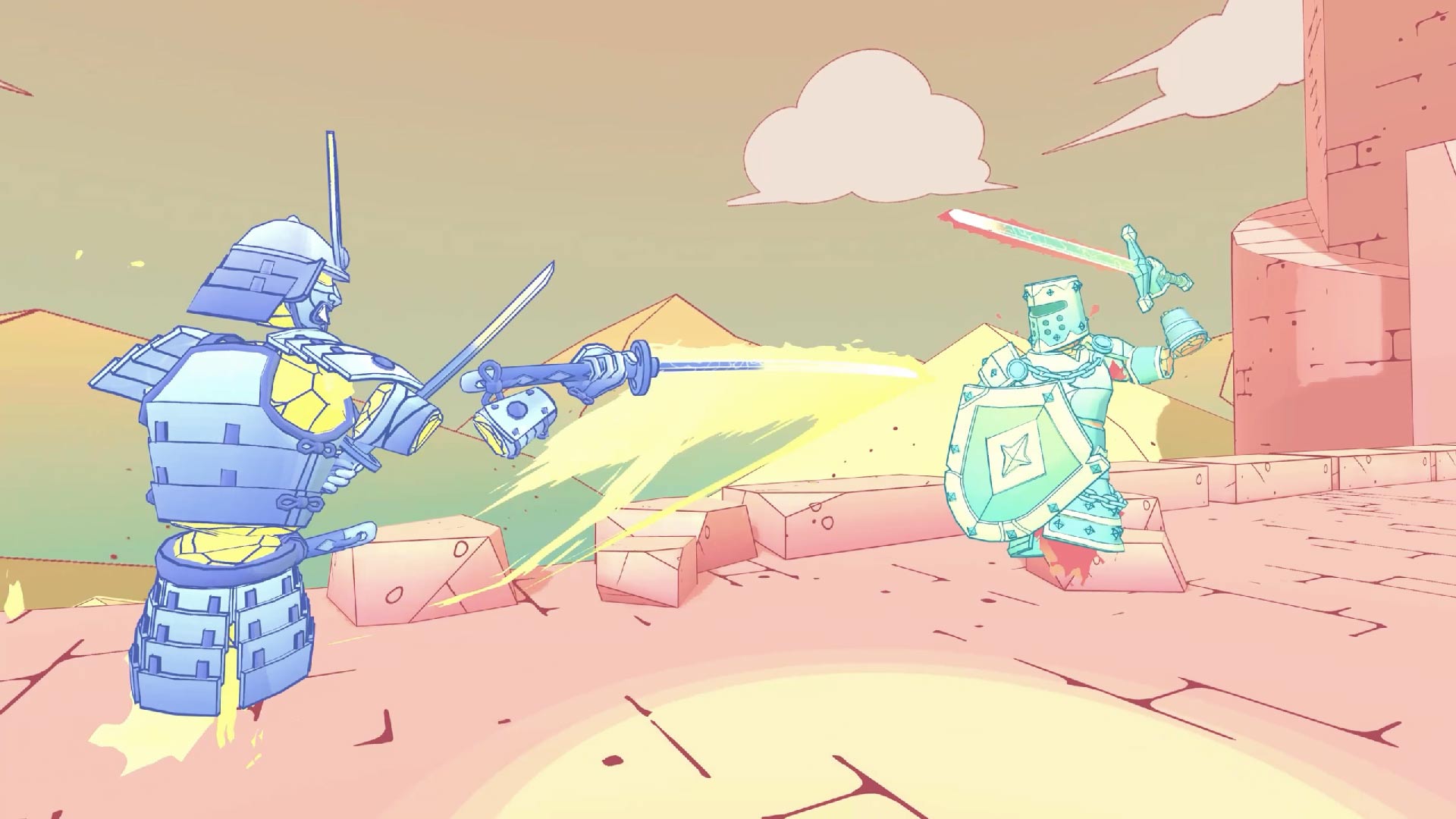This vibrant, digital illustration, potentially a concept for a video game, depicts a dramatic scene on a large, brick wall resembling the Great Wall of China. The stone surface and brick structures, colored in light red, extend into the background, where a castle turret is visible on the far right. Floating above the wall are two spectral figures dressed in contrasting medieval armors, devoid of legs and bodies, giving them a ghost-like, robotic appearance. 

On the left, a figure in traditional samurai armor, characterized by intricately arranged metal plates and an elaborate helmet, wields a flaming samurai sword. This figure contrasts with the knight on the right, who is clad in classic European armor, equipped with a large shield and a sword. Both figures seem to hover slightly above the ground as they engage in combat amidst the stone environment. The visual composition is rendered in a simple, yet striking, animated style with bright, Easter-like color palettes, including shades of blue, green, pink, and red. The sky above features large, light red clouds that add a dramatic flair to the scene, possibly illuminated by the yellow rays from the fight. The image evokes a sense of mystique and excitement, making it an intriguing piece possibly intended for a video game concept.